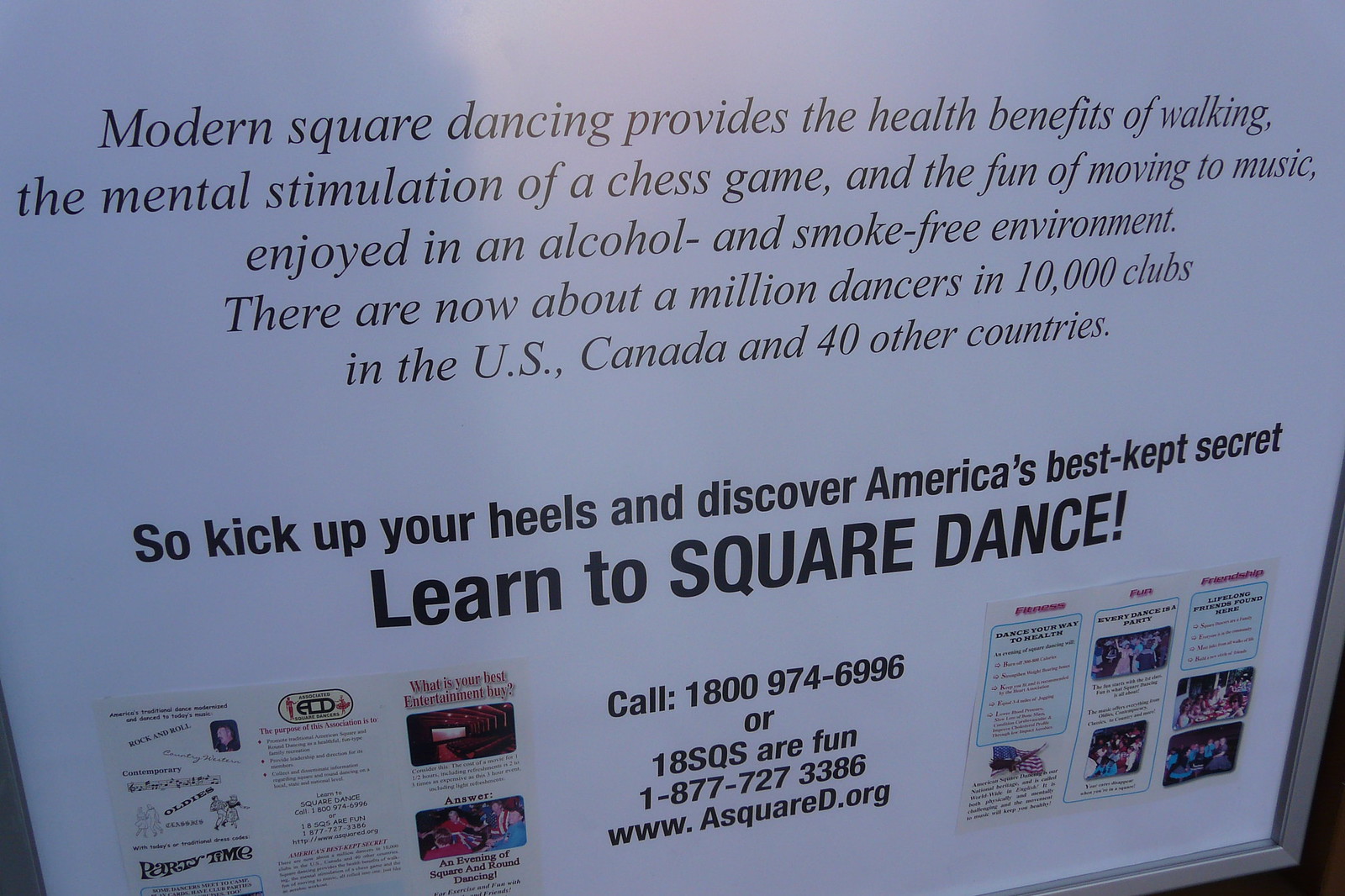This horizontally aligned rectangular image appears to be a framed poster, indicated by the visible bottom and right sides of a silver frame. The poster features a centered title at the top that states: "Modern square dancing provides the health benefits of walking, the mental stimulation of a chess game, and the fun of moving to music. Enjoy it in an alcohol and smoke-free environment. There are now about a million dancers and 10,000 clubs in the U.S., Canada, and 40 other countries." Below this text, in bold, larger print centered in the middle, it urges: "SO KICK UP YOUR HEELS AND DISCOVER AMERICA'S BEST-KEPT SECRET. LEARN TO SQUARE DANCE!" The phrase "LEARN TO SQUARE DANCE" is highlighted in uppercase black letters with an exclamation mark. Centered below this, the poster provides a contact number, "1-800-974-6996 or 1-8-SQS-R-FUN" and an additional number, "1-877-727-3386," followed by the website "www.asquared.org." Flanking this contact information are smaller posters or brochures, each consisting of three columns, with a mix of images and text, likely related to square dancing.